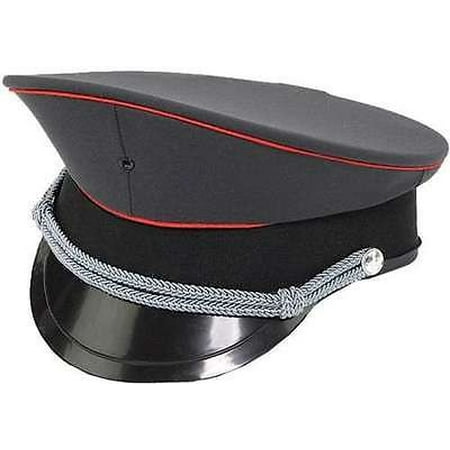This is a detailed color photograph of a military-style hat prominently displayed against a plain white background. The hat features a striking shiny black visor at the front, slightly angled towards the lower left corner, with light reflecting off its surface. Above the visor, a double silver chain or cord stretches across the front of the hat, held in place by silver buttons on each end. The body of the hat is primarily composed of dark gray or charcoal cloth, with a distinct red stripe or piping running near the top edge, about a half inch from the top. Below the red piping, the hat has a darker black band, possibly a different texture suggestive of black felt. The overall design is clean and austere, highlighting the hat's military influence through its structured form and color scheme of gray, red, silver, and black.